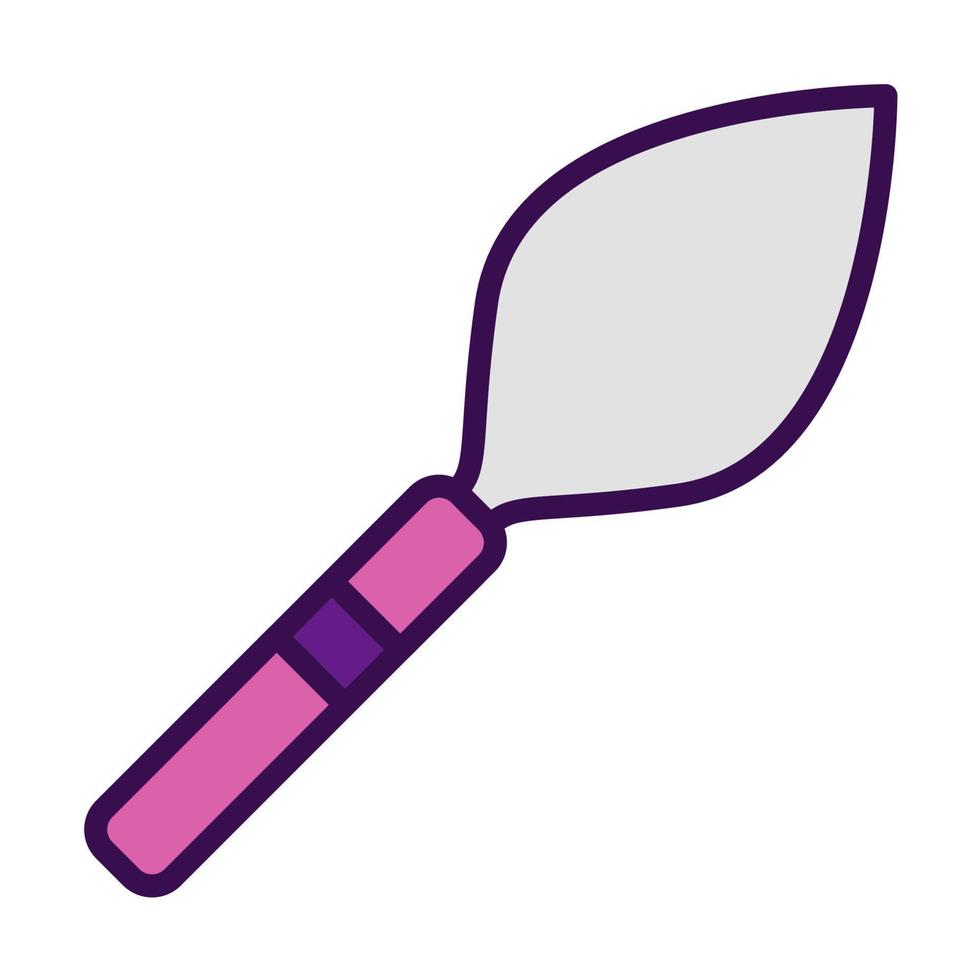The image is a simple vector illustration with a white background, depicting a tool with an angled handle pointing towards the bottom left and the head pointing towards the top right. The tool appears to be a cartoonish interpretation, much like something a child would draw. The handle is cylindrical and pink with dark purple borders. It features two horizontal lines filled with a violet color. The top part of the tool is shaped somewhat like a small gardening shovel or spoon and is light gray in color. The overall appearance is clean and minimalistic, with both the handle and the head uniformly outlined in dark purple.